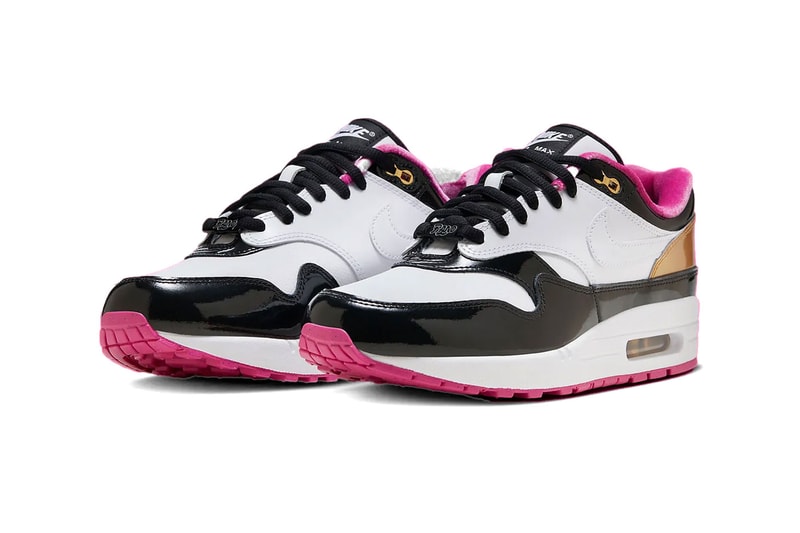This is a detailed image of a pair of brand-new Nike Air Max sneakers taking up the entire frame against a white background. The sneakers feature a vibrant combination of colors: primarily white with black accents, bright pink highlights, and small touches of gold. The shoes are oriented pointing slightly to the left, showcasing more of the front than the sides. The shoelaces are black, the inner lining and the bottoms are a striking pink, and both the heel and one of the shoelace eyelets have hints of gold. The Nike Swoosh logo blends subtly into the white areas of the shoes. The sneakers have thick soles, a shiny, unworn appearance, and they seem to be designed for women. The white background is devoid of any other elements, making the sneakers the clear focal point of the photograph.